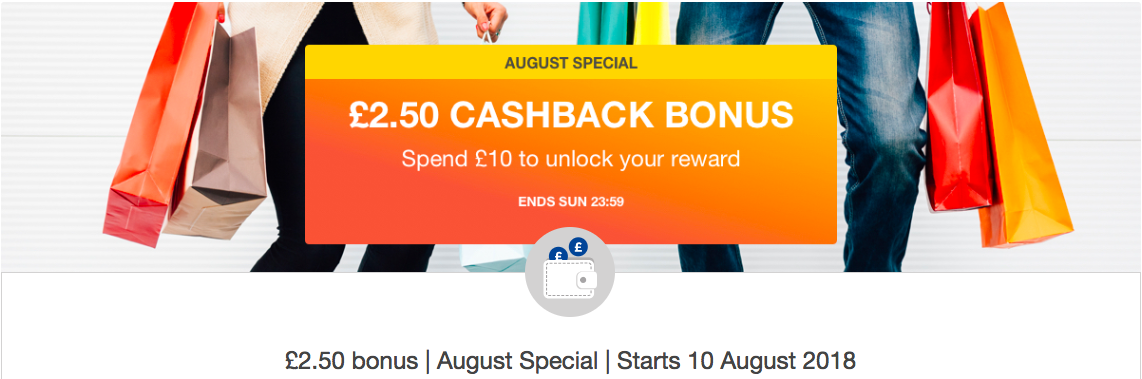Screenshot of a Webpage Advertising August Special Cashback Bonus

The screenshot displays a webpage with a white background. At the bottom of the image, there is a black text banner with moderate font size, stating "£2.50 bonus" accompanied by a vertical line that reads "August Special." Another vertical line indicates the date "10 August 2018."

To the left, a woman is partially visible, wearing black leggings and a thin white jacket. She is holding a pink and orange bag in her right hand. Next to her, on the right, stands a man in slightly faded blue jeans, holding a yellow bag in his left hand.

Central to the image is a large, rectangular advertisement. The top section of the advertisement is yellow with the text "August Special" in black font. Below, the background shifts to orange and reads "£2.50 cashback bonus" in a larger font. Beneath this, additional text in a smaller font states, "Spend £10 to unlock your reward. Ends Sunday, 2359."

The image provides a clear depiction of a promotional offer with visually appealing colors and targeted information.